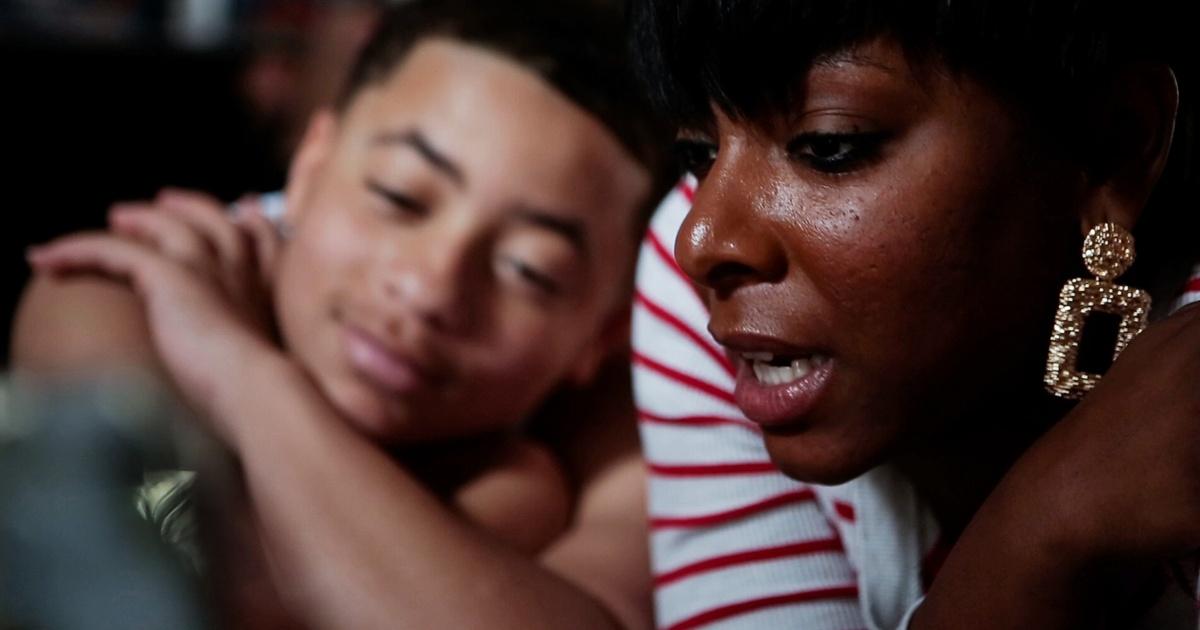The photograph portrays an African-American woman and a younger male lying on their stomachs, propped up on their elbows. The woman, who has dark brown skin and short hair visible from a cropped angle, wears a striking white and red striped long-sleeved t-shirt and large, rectangular gold earrings reminiscent of belt buckles. She appears to be mid-conversation, possibly talking on a speakerphone out of frame. The younger male beside her, approximately 15 years old with a close-cut haircut and slight facial hair, rests his chin on his arm and smiles faintly. He's out of focus and wears a tank top, leaning slightly towards the woman. The intimate setting features warm colors and high contrast, bringing out the textures of the woman's earrings and shirt, while the blur adds a sense of depth to their interaction.